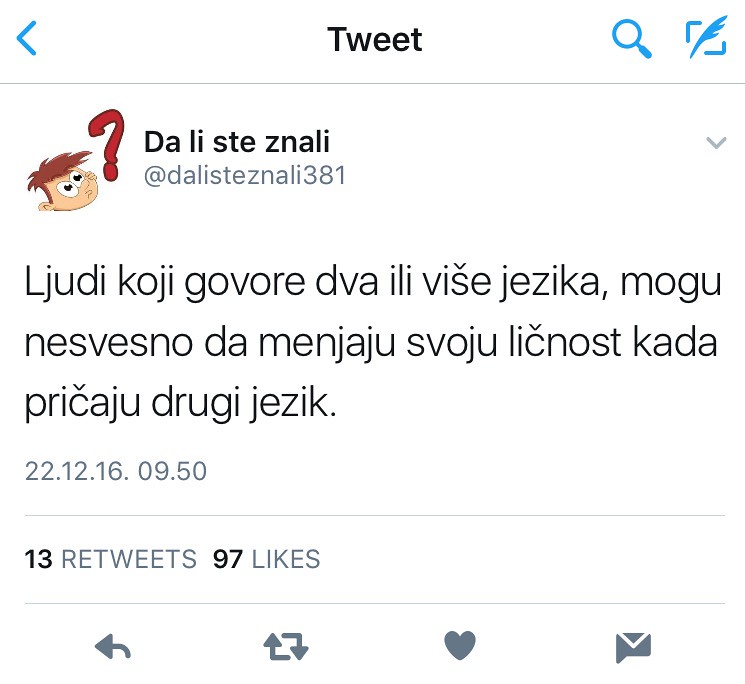This is a detailed screenshot of a tweet from Twitter, displaying a white background with a top navigation bar. On this bar, a blue back icon, a black 'Tweet' label in San Serif font, and two icons—a blue magnifying glass for search and a feather quill for writing—are visible at the top right. The tweet, written in a foreign language and consisting of three lines of text likely in Helvetica font, is by a user with the handle @DallasDinsNally381. Their profile picture is a cartoon image of a character with beige skin, fluffy brown hair, and large eyes, next to a red question mark. The tweet shows the date 22-12-16 and time 9:50, with 13 retweets and 97 likes. Below the tweet, icons for a back arrow, retweet, heart, and message, all in gray, are present.